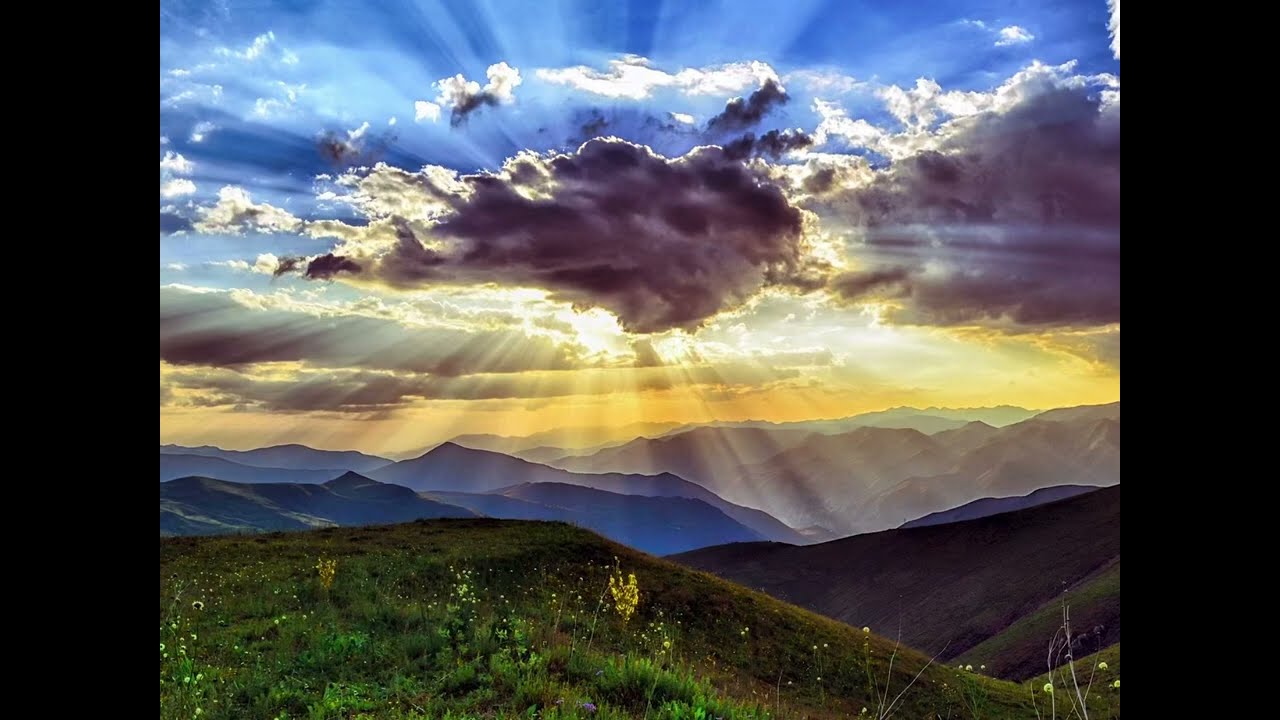In this detailed and vibrant artwork, we see an exquisite outdoor scene featuring a lush, grassy hilled landscape dotted with yellow wildflowers. The foreground is rich with various lengths of green grass and some scattered weeds. Stretching into the distance, the rolling hills transition into a majestic blue and gray mountain range partially shrouded in mist. Dominating the sky is a dramatic display of clouds and sunlight. At the top, the sky is a clear, vivid blue with scattered white clouds. The visual centerpiece is a massive dark gray cloud tinged with purple and illuminated by the sun, which is positioned behind it. This cloud is flanked by another large rain cloud on the right. Golden rays of sunlight pierce through the clouds, spreading in every direction—north, south, and west. The sky transitions to a warm orange hue around mid-image, creating a stunning contrast with the cool tones of the mountains below. This scene is captured in broad daylight, showcasing the incredible detail and beauty of nature’s landscape.